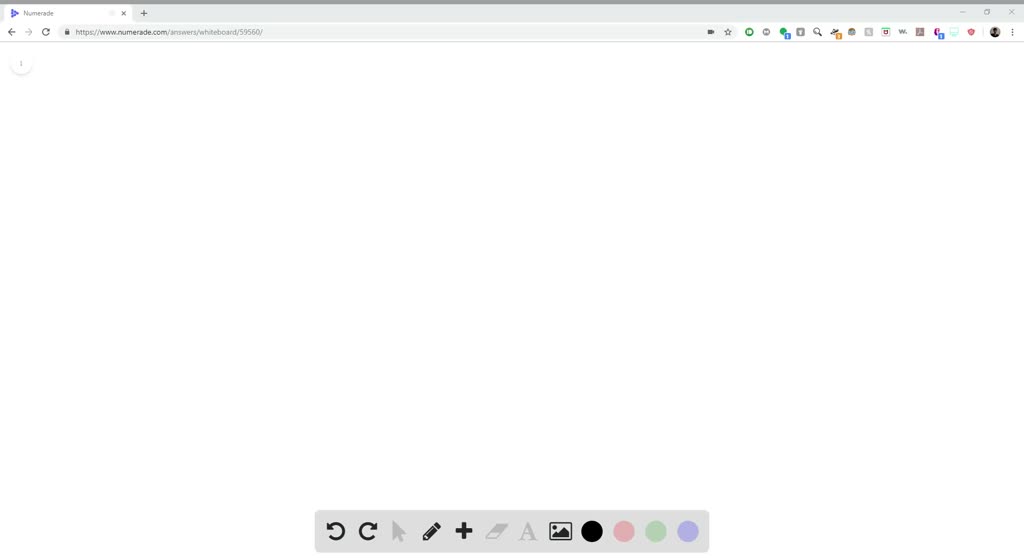This image is a screenshot of a webpage from the URL https://www.numerate.com/.answers/.whiteboard/.59560/, which seems to belong to a platform or application called NumerAid. 

At the top of the image, there is a grey navigation bar. On the left side of the bar, there's a blue triangle-shaped tab with the word "NumerAid" written next to it. Adjacent to this are navigation controls including back and forward arrows, a reload arrow, and the website address mentioned earlier. 

The main area of the screenshot appears mostly blank, but on closer inspection, there is a partially visible grey round button with a faint line in the center on the left side.

On the right edge of the screen, a cluster of small, somewhat blurry, multi-colored icons is visible. These include icons with blue message symbols next to them, green circles, greyed-out icons, and one with a yellow message symbol. 

Additionally, at the far left edge, there is an icon depicting a head and shoulders silhouette outlined in black against a grey background, accompanied by a hamburger menu icon.

Toward the bottom of the screenshot, there is a light grey dock containing various tool icons. These include back and forward buttons, a greyed-out arrow, a pencil icon, a plus icon, and an eraser icon that is also greyed out. Also present are a greyed-out text icon and a picture icon. The dock features four round buttons that are black, pink, green, and purple respectively; the pink, green, and purple buttons appear muted or greyed-out. This suggests that the dock is likely part of a drawing menu, indicating that the webpage may offer interactive drawing or annotation capabilities.